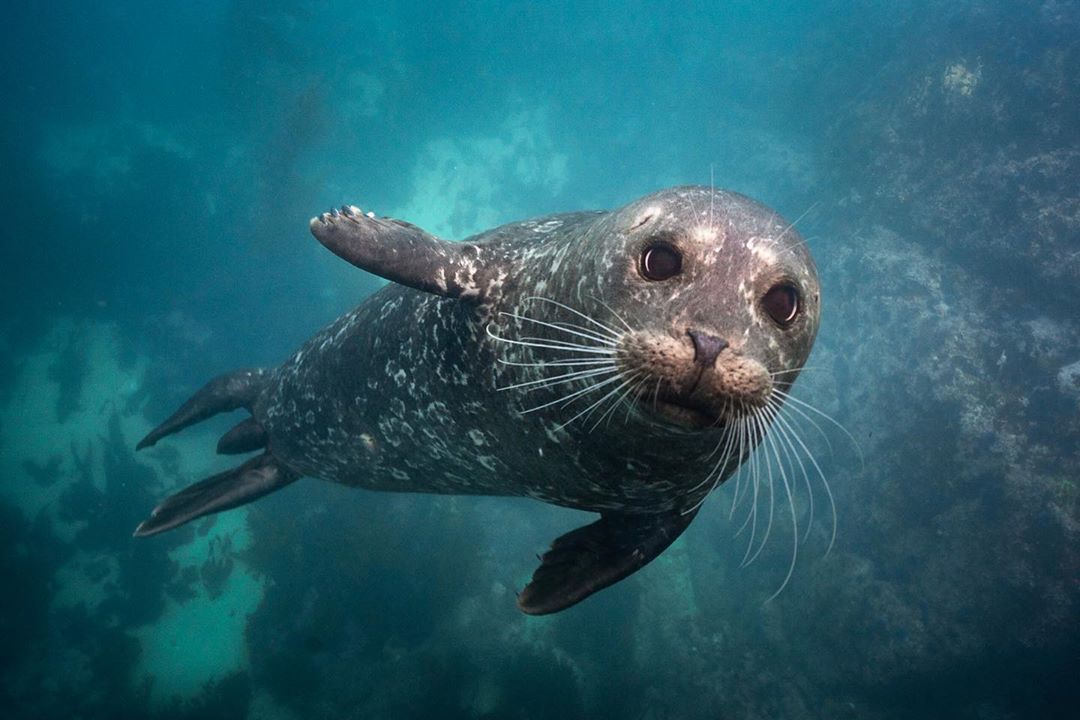In the image, we see a young sea lion swimming underwater, staring directly at the camera with large, dark eyes. Its snout, resembling a peanut with holes, is adorned with long, white whiskers that give it a distinct and cute appearance. The creature's skin is brownish-dark with small white spots and patches of black blubber, while tiny flippers extend back from its body. It swims gracefully through the greenish-tinted water, which slightly obscures the view of its surroundings. In the background, we can observe rocky formations with various markings and flowing sea plants, indicating the sea lion is in its natural habitat. The photograph is focused on the sea lion, which is positioned diagonally in the center, making it the main focal point of the scene.